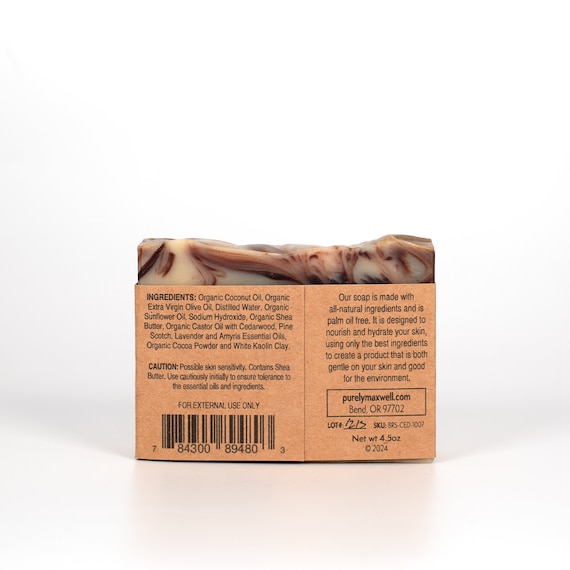The image depicts a luxury bar soap, positioned centrally on a white surface. The soap is partially wrapped in a paper label that reveals its all-natural, palm oil-free composition designed to nourish and hydrate the skin. The soap's exposed top edge is jagged, as if it was broken from a larger piece. The label lists ingredients such as organic coconut oil, organic extra virgin olive oil, distilled water, organic sunflower oil, sodium hydrocarbon, organic shea butter, organic castor oil, cedar wood, pine scotch, lavender, and amethyst essential oils, organic cocoa powder, and wheat caroline clay. The soap itself appears in shades of white, brown, and black, with reddish-pink hues. Additional details on the label include an external use warning, a barcode, and the manufacturer’s information from Bend, Oregon, as well as a website (purelymaxwell.com). The soap casts subtle shadows on the white background, adding depth to the image.